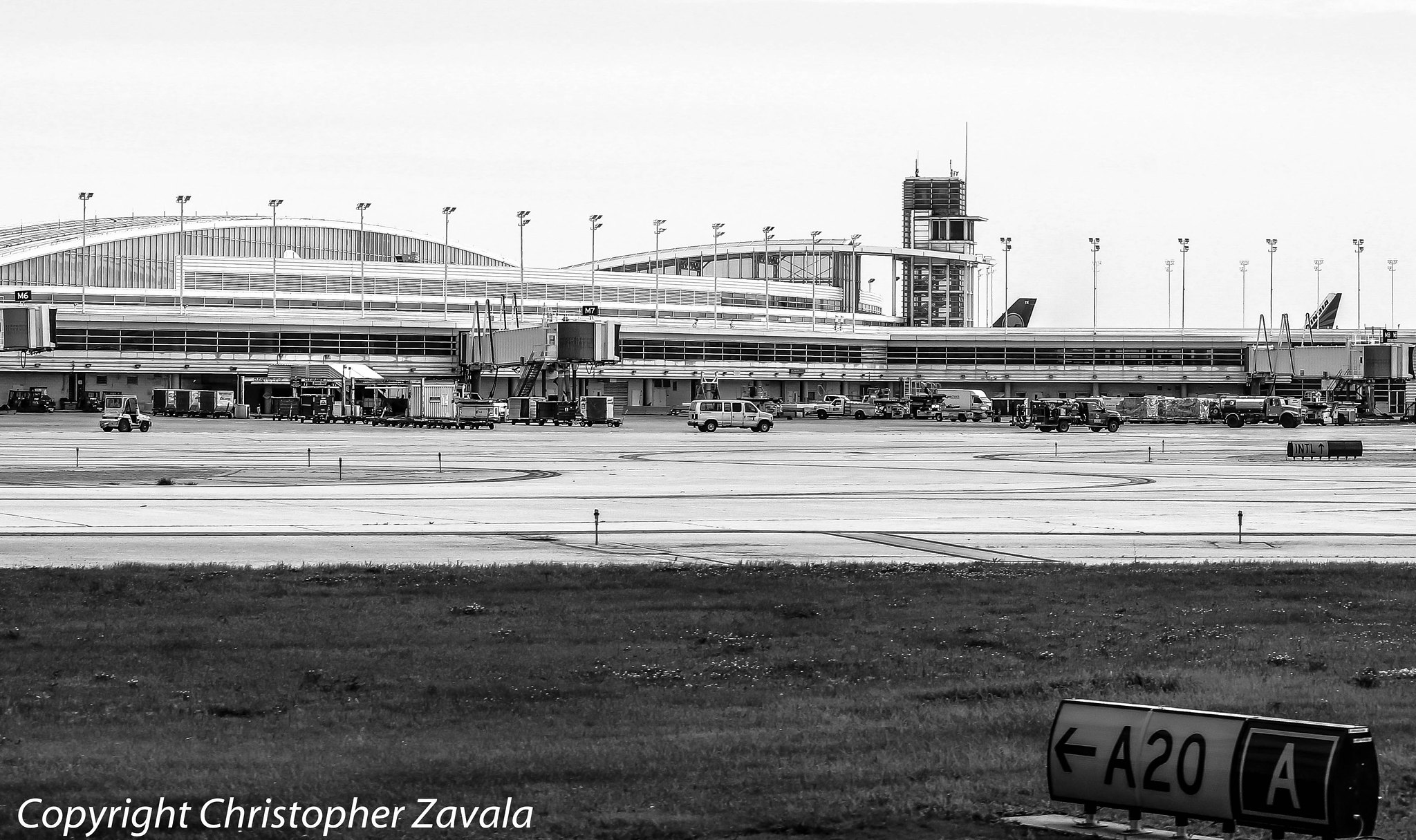This black-and-white photograph by Christopher Zavala captures a bustling scene at Dallas-Fort Worth Airport (DFW). Prominently featuring the baggage handling area, the image showcases various American vehicles, including fuel trucks, fire trucks, and the small vehicles that pull trains of baggage carts. The central focus is on the vehicles and the airport infrastructure, with a clear runway marker labeled "A20A" positioned in the foreground on the bottom right. The airport's curved rooflines and distinctive window shapes are visible in the background, along with the tails of aircraft peeking over the buildings. This detailed composition vividly portrays the organized chaos of airport logistics and provides a nostalgic glimpse into DFW's operational environment.